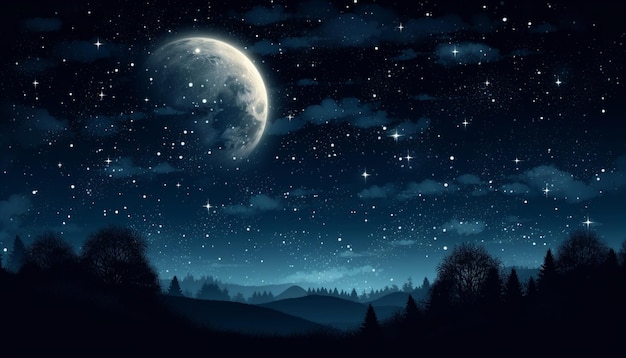This is a digital piece of graphic art illustrating a mesmerizing night sky. The scene captures a large, glowing white moon that dominates the horizon, radiating a soft light. The sky above is a rich, dark blue with hints of a green-blue hue in the distance, peppered with numerous white stars. Silhouetted clouds, taking on a translucent whitish quality, float across the sky, adding to the ethereal ambiance. Below, rolling hills stretch into the distance, their light and dark blue silhouettes blending seamlessly with the landscape. Scattered along these hills are black silhouettes of trees, contributing to the serene yet striking composition. The entire image exudes a calm and otherworldly beauty, showcasing the tranquil splendor of a moonlit night.